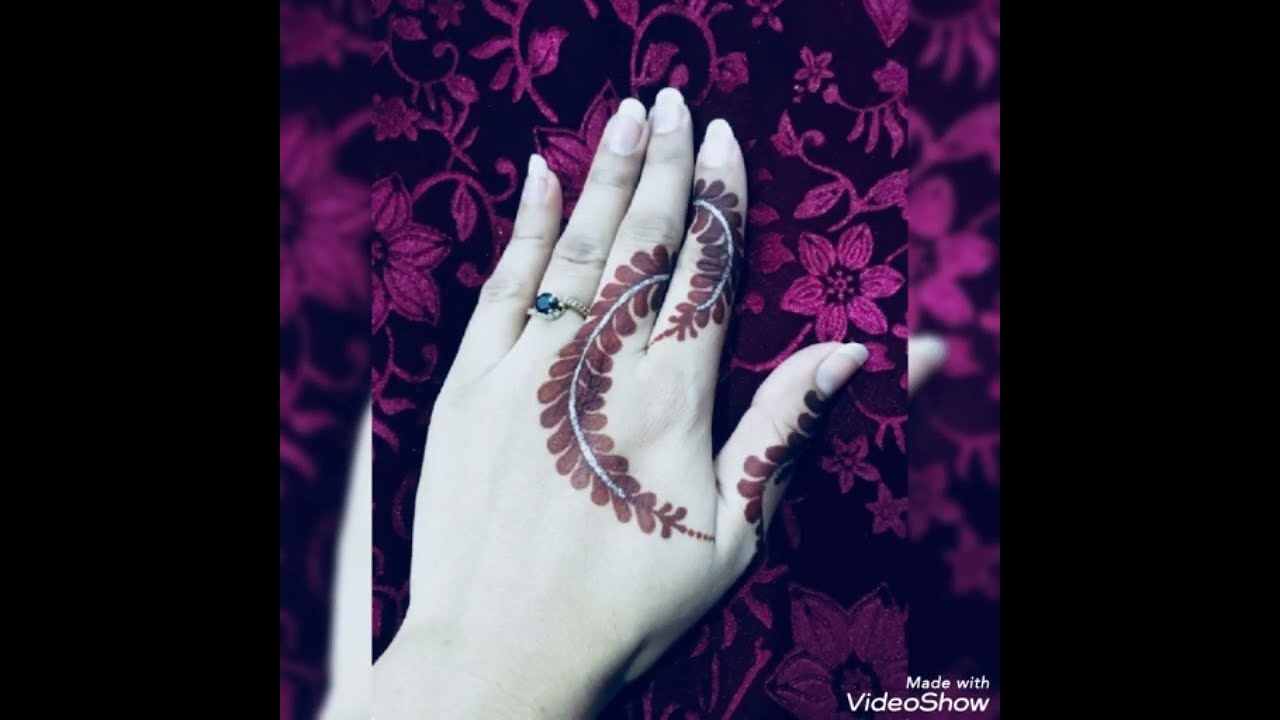The image features a prominently positioned woman's left hand adorned with a detailed, possibly henna, design resembling leaves that wrap around her index finger, curl across her knuckles, extend to her thumb, and cross to her middle finger. Her fingernails are long and unpainted, and she wears a striking sapphire set in a gold ring on her ring finger. The background is a richly textured purple floral pattern, likely a tablecloth or fabric, giving the setting an elegant and artistic feel. The photo is flanked by two slightly out-of-focus and enlarged panels on the left and right sides, mirroring portions of the main image. At the bottom right corner, there is text that reads "Made with VideoShow," suggesting that the image might be part of an advertisement or a creative project.